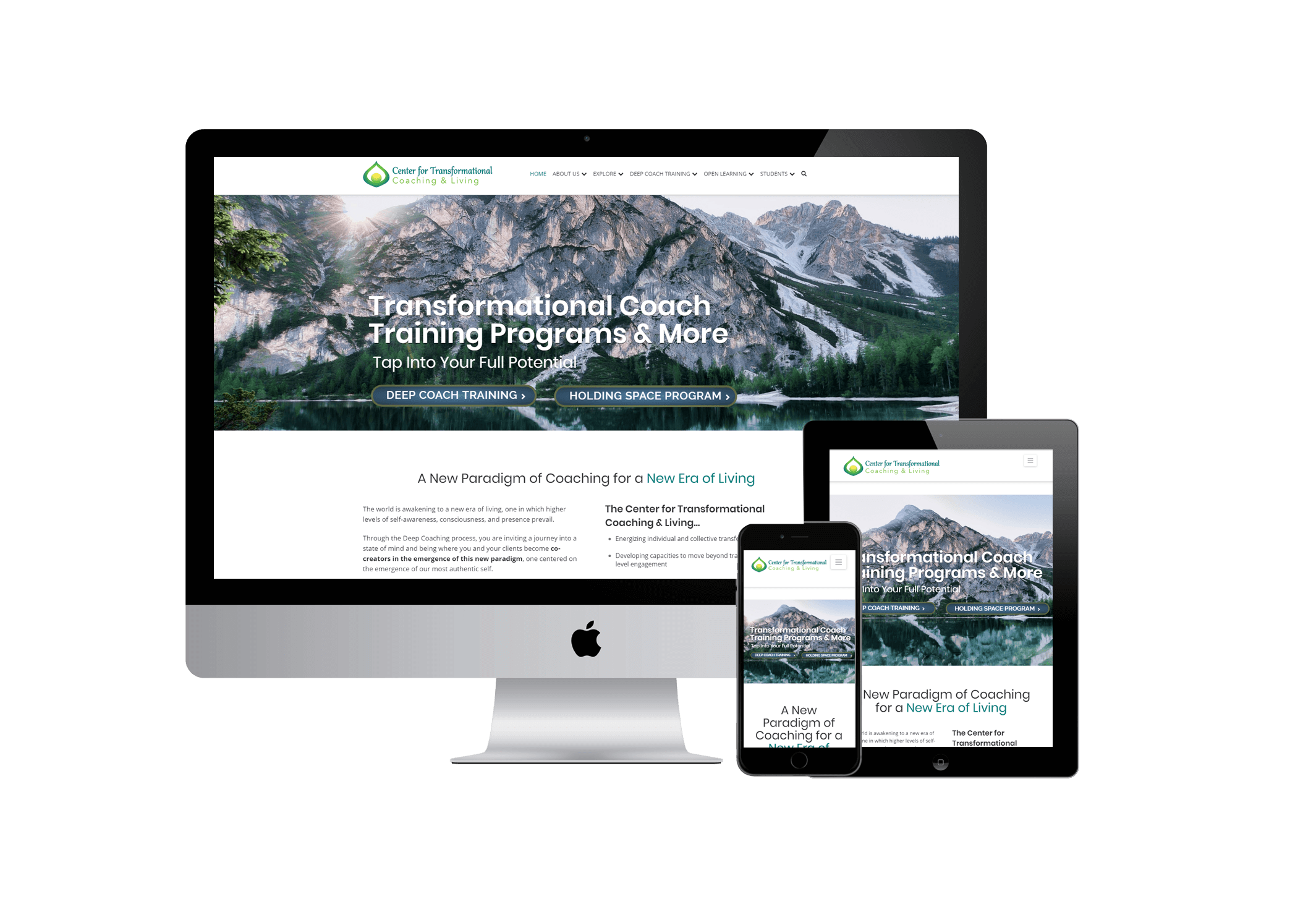Three devices—an Apple computer flat-screen monitor, a smartphone, and a tablet—display the same website, illustrating its responsive design. The silver Apple monitor, distinguished by the iconic black Apple logo at its bottom center, serves as the backdrop. In front of the monitor, both the smartphone and tablet, each framed by a black border, showcase the website's adaptive layout.

The webpage header reads "Center for Transformational Coaching and Living," followed by navigation links: Home, About Us, Explore, Deep Coach Training, Open Learning, and Students. A stunning photograph of a mountain range adorns the background, complementing the text "Transformational Coach Training Programs and More" and the empowering message "Tap into your full potential. Deep Coach Training, Holding Space Program."

Below this, a visionary statement is partially visible: "A New Paradigm of Coaching for a New Era of Living. The world is awakening to a new era of living, one in which higher levels of self-awareness, consciousness, and presence prevail. Through the deep coaching process, you are invited on a journey into a state of mind and being where you and your clients become co-creators in the emergence of this new paradigm, one centered on the emergence of our most authentic self."

The footer starts with "The Center for Transformational Coaching and Living" and continues with "Energizing Individual and Collective," but the rest of the text is cut off. The subsequent line, "Developing Capacities to Move Beyond," is also truncated, hinting at a deeper narrative on the website.